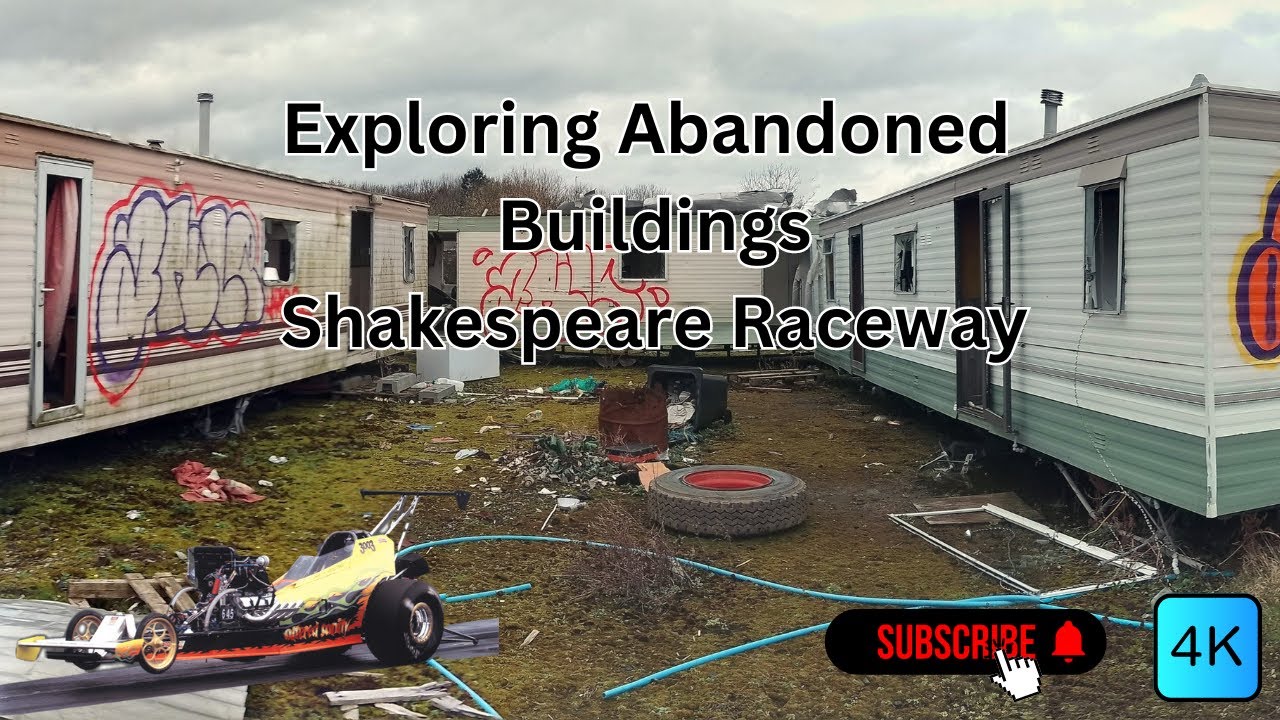This image, likely a YouTube video thumbnail, depicts a desolate and abandoned area called Shakespeare Raceway. The focal point consists of three trailer homes configured in a U-shape, creating an enclosure around a central area filled with trash and debris. The trailer on the left is dirty and covered in red and purple graffiti, while the one in the back, perpendicular to the others, also displays prominent red graffiti. The trailer on the right appears slightly cleaner, painted white with a green stripe, but with broken windows and an open door. Scattered across the ground are numerous items of debris, including an old tire with a red ring, a rusted barrel, an overturned trash can, a blue hose, a window frame, cinder blocks, and what looks like an old refrigerator.

Additional visual details include a superimposed or photoshopped image of a race car in the bottom left corner, hinting at the raceway theme. The sky is cloudy, adding to the abandoned and rundown atmosphere. Centrally displayed text reads, "Exploring Abandoned Buildings, Shakespeare Raceway." In the bottom right corner, an icon for "4K" is set in a rounded blue square, and nearby, a black oval with red text and a bell icon prompts viewers to "subscribe," indicating this is part of a video content aimed at an online audience.